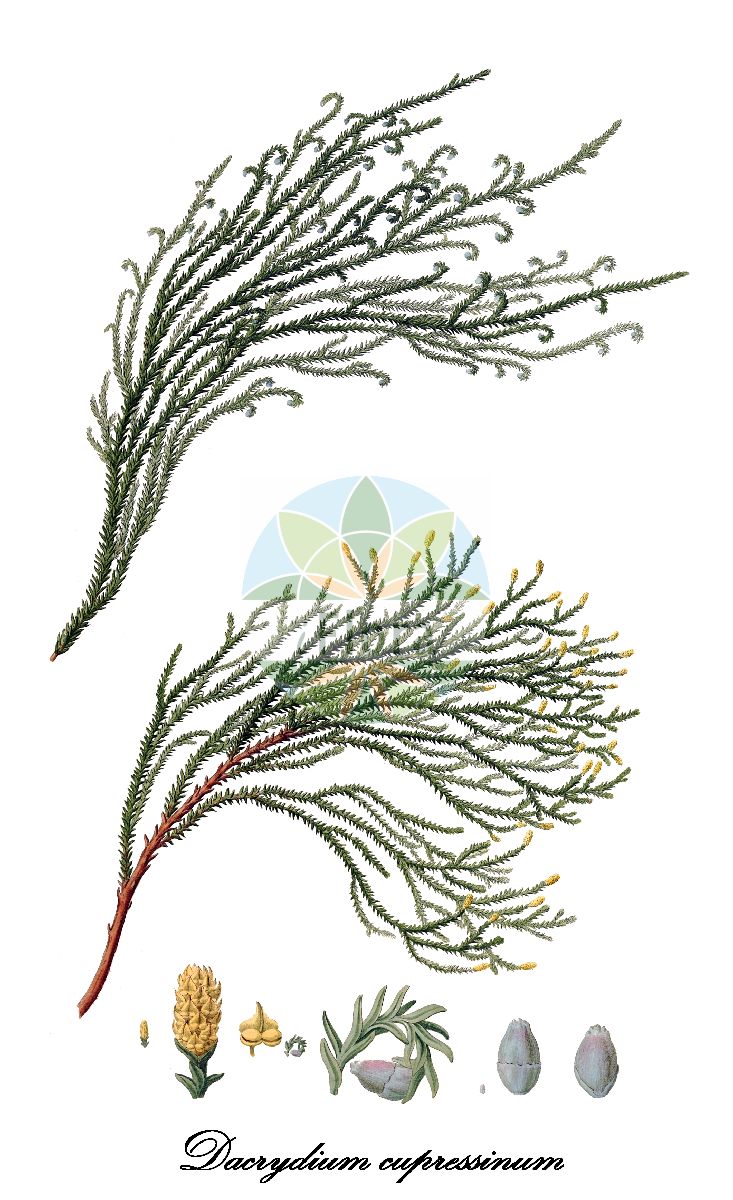This digital illustration, likely created with computer graphics, depicts two types of plants against a white background, flowing upward from the left to the right. The plant on the left features a purely green stalk with a small wooden break at the base, while the plant on the right exhibits a gradient from a cool brown wooden stalk to green as it ascends. Both plants are detailed with prickly leaves that resemble spikes. The illustration includes a half-circle with a rotating green flower at its center, marked by a yellow core and encircled in blue. Between the two plants, additional cross-sections reveal their seed structures and green stalk segments, accompanied by cursive text beneath that likely denotes the plant's Latin name, Daccharidium scopressinum. The bottom part of the design also includes visual breakdowns of seeds and flowers, suggesting this image serves as a detailed design template. Notably, a faint watermark adorns the image, signifying its professional or artistic origin.